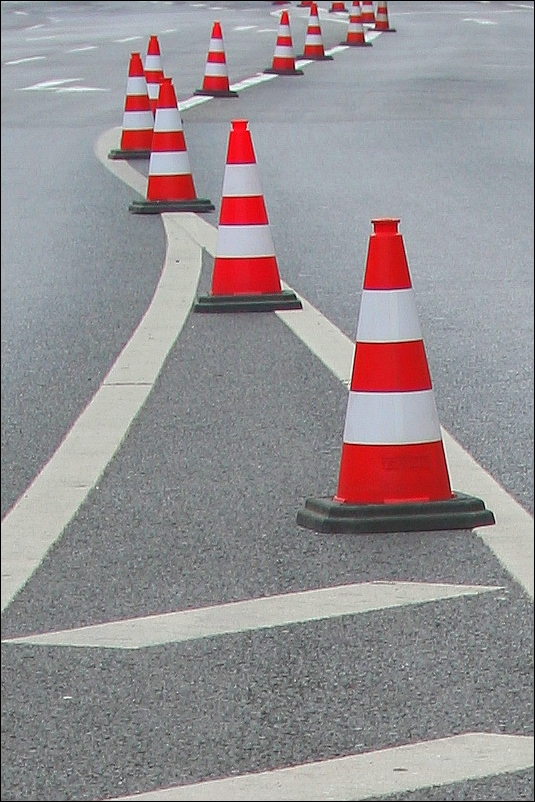A detailed view of a paved street showcases a triangular section of white paint starting from the foreground and extending to the middle of the image. Within the triangle, two horizontal white dashes are clearly visible. To the right of the triangle's apex, the white line curves off and then extends further up to the left. Scattered across the painted lines are several traffic cones. Most cones align with the lines, although two are positioned inside the triangular section. Each cone features a black base and alternating bands of orange and white, culminating in an orange tip at the top.